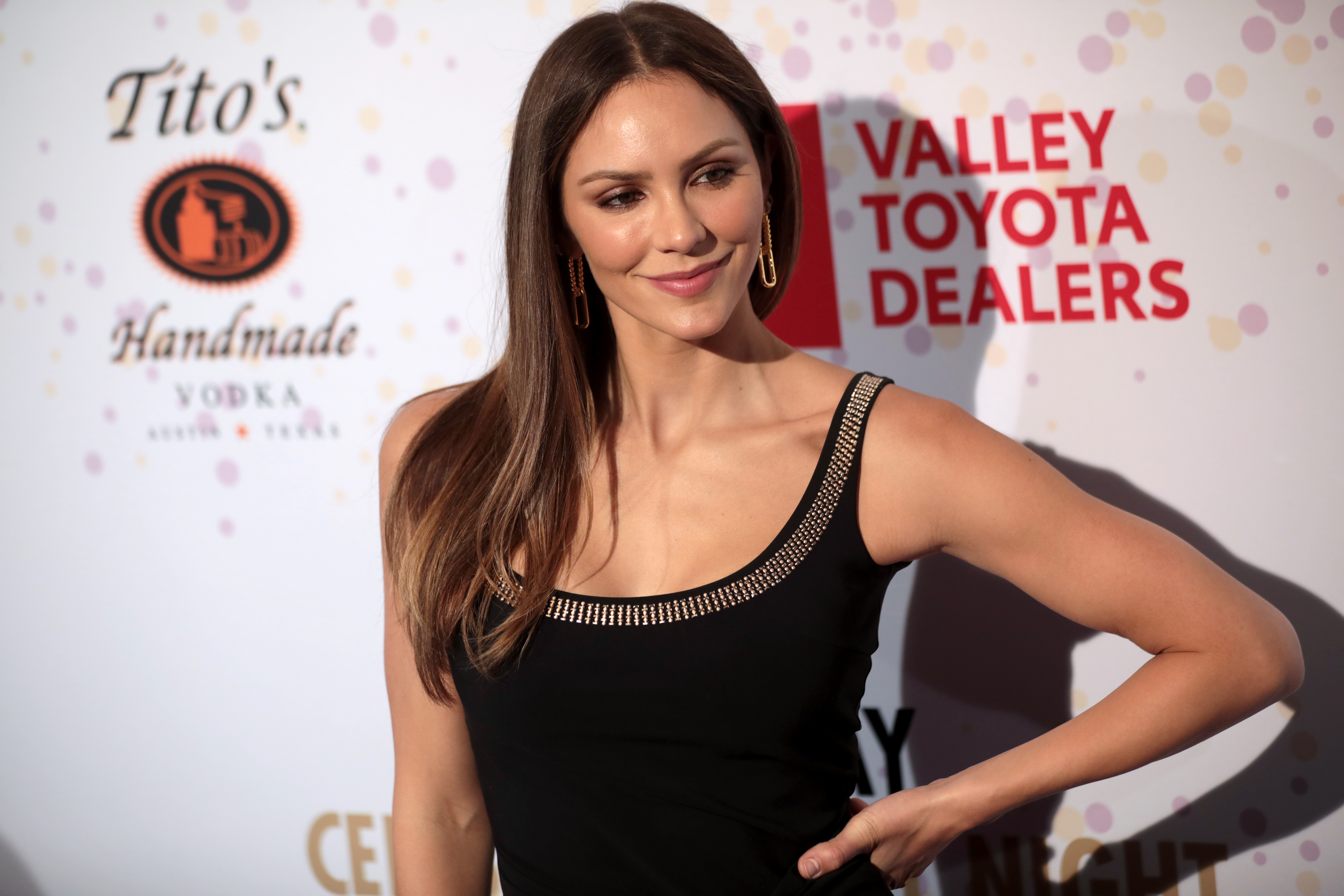The image captures a white singer-actress posing at a celebrity event, likely on a red carpet, with her left hand confidently placed on her hip. She sports long brown hair that cascades down to her breasts, complemented by gold oval earrings that dangle like chains. Her attire features a black garment with intricate beading and a low neckline, accentuated by a gold or metal trim around the edges and straps. The background showcases a sponsor's banner dotted with logos and text, including prominent brands like "Tito's Handmade Vodka" and "Valley Toyota Dealers" in red lettering, partially visible behind her. The signage is festooned with a vibrant array of colors such as pink, peach, black, white, gold, red, purple, yellow, orange, and a hint of tan. She has a glowing tan and wears pinkish lipstick while smiling and engaging with the camera, adding to the professional and polished vibe of the photograph.